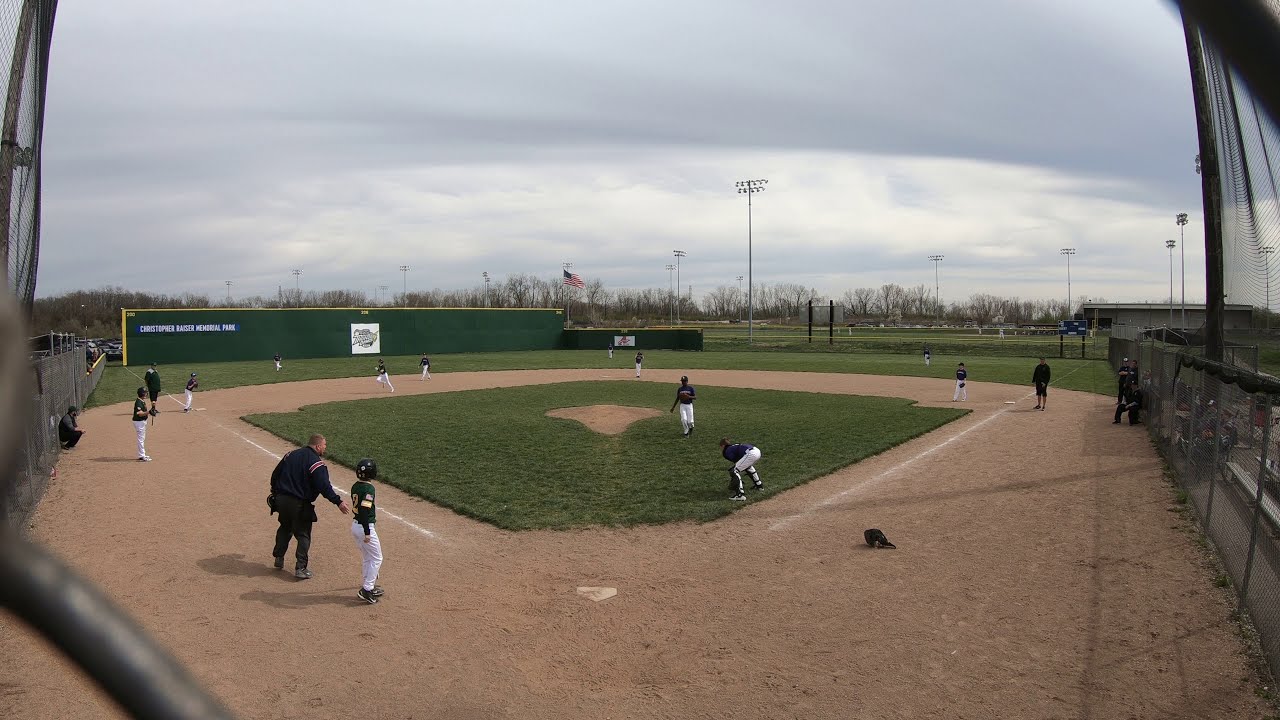The photograph captures an outdoor daytime baseball game at what appears to be a Little League field, possibly Christopher Rager Memorial Park. The image is taken from the perspective behind home plate, looking through a chain-link fence. The scene features a standard baseball diamond with a white home plate, white baselines, a grass infield, and a brown pitcher's mound. 

Several players are visible on the field, with some wearing green jerseys and white pants, while others are in blue jerseys and white pants. The distinction between the teams is blurred due to the similar color schemes. A player is seen running towards third base while the catcher, positioned on the grassy infield, appears ready to throw the ball. There is an adult in black, possibly an umpire or coach, standing near home plate. 

In the background, a green fence encloses the outfield, which is higher on the left side than the right. Beyond the fence, an American flag flies from a tall pole, and tall floodlights, which are off, indicate that the game is taking place during the day. Sparse trees and a parking lot with several vehicles can be seen further in the background. The sky is heavily overcast with gray and white clouds, creating a backdrop that emphasizes the outdoor setting. The field is bordered by a combination of chain-link fencing and solid walls in certain areas, adding to the typical look of a community baseball field.